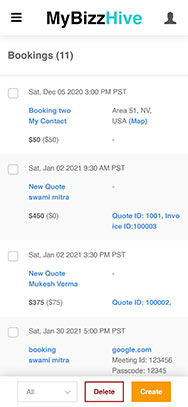The image features a user interface with a clean white background. At the top, there is a hamburger icon followed by the text "My Biz Hive" in blue. A black profile icon is visible next to the text, which shows "(Bookings: 11)".

Below are several list items, each prefixed with a checkbox. The first notable entry reads:

- Saturday, December 5th, 2020, at 3:00 PM PST
    - Contact: [Click here](#) (in blue)
    - Fee: $50 (in parentheses)
    - Location: Area S1, NB, USA (with the term "S1" being somewhat illegible)
    - Map: [View Map](#) (in blue)

Another entry is structured as follows:

- Saturday, January 2nd, 2021, at 9:30 AM PST
    - New Quote: Swami Mitra
    - Fee: $450 (in parentheses)
    - Zero dollars quote (in parentheses)
    - Quote ID: 1001001
    - Invoice ID: 100003

There is an additional entry for the same date:

- Saturday, January 2nd, 2021, at 3:30 PM PST
    - New Quote: Makisha Verma